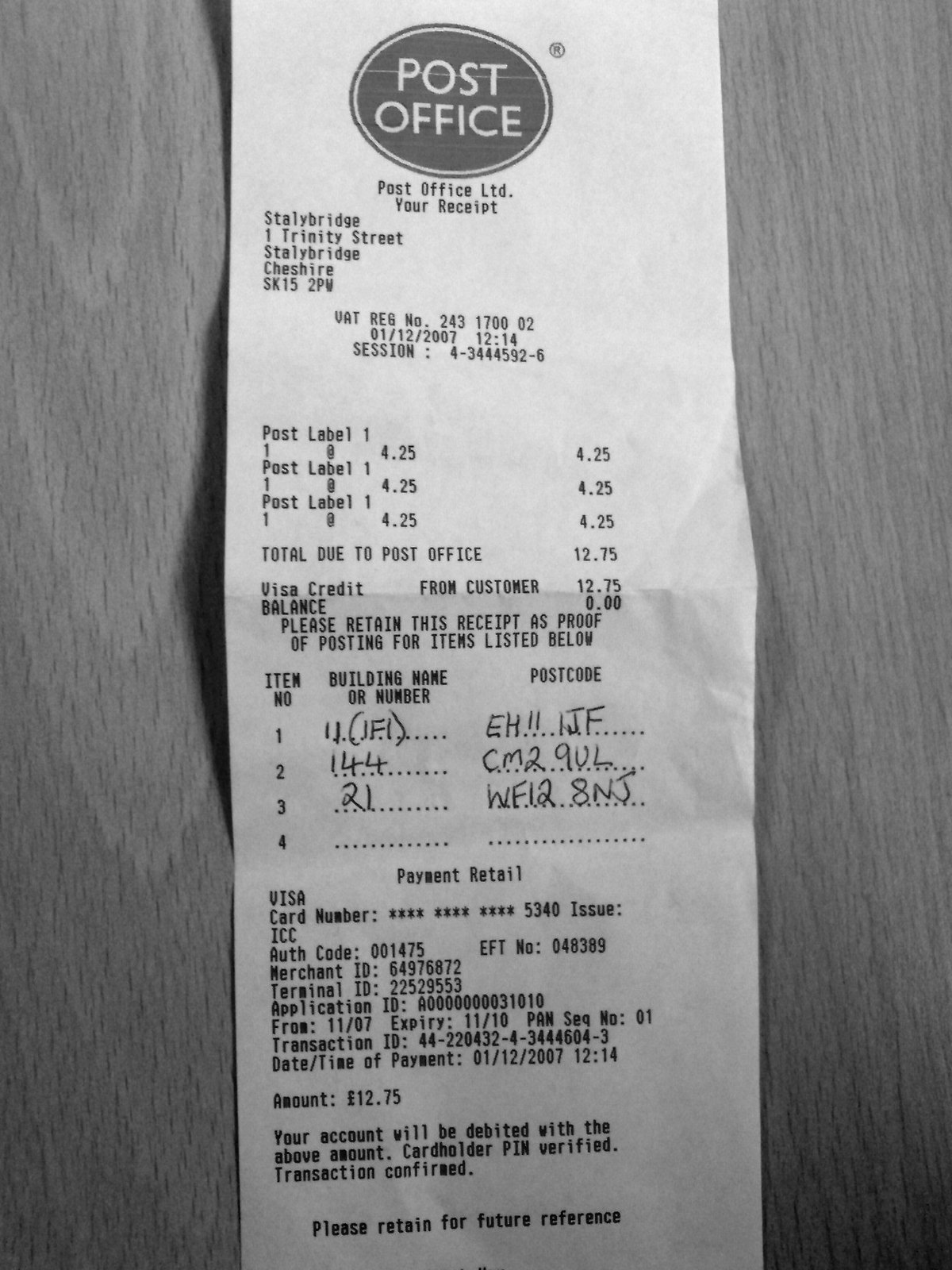A detailed and cleaned-up caption for the described image could be:

"The image displays a folded and creased white paper receipt from the post office, positioned vertically within a gray oval border, with 'POST OFFICE LTD' and 'Your Receipt' prominently printed in white capital letters at the top. The receipt is issued by the Stalybridge branch located on Trinity Street, Stalybridge, Cheshire, with a specific postcode listed. The transaction details indicate that the owner mailed three packages, each with an individual cost of $4.25. The receipt itemizes the destinations, listing building names and postcodes for each mailed package. At the bottom, there is a note about a personal payment retail transaction. Additional handwritten notes are visible in the lower section. The entire setup is photographed against a gray wood grain countertop, adding texture to the overall presentation."